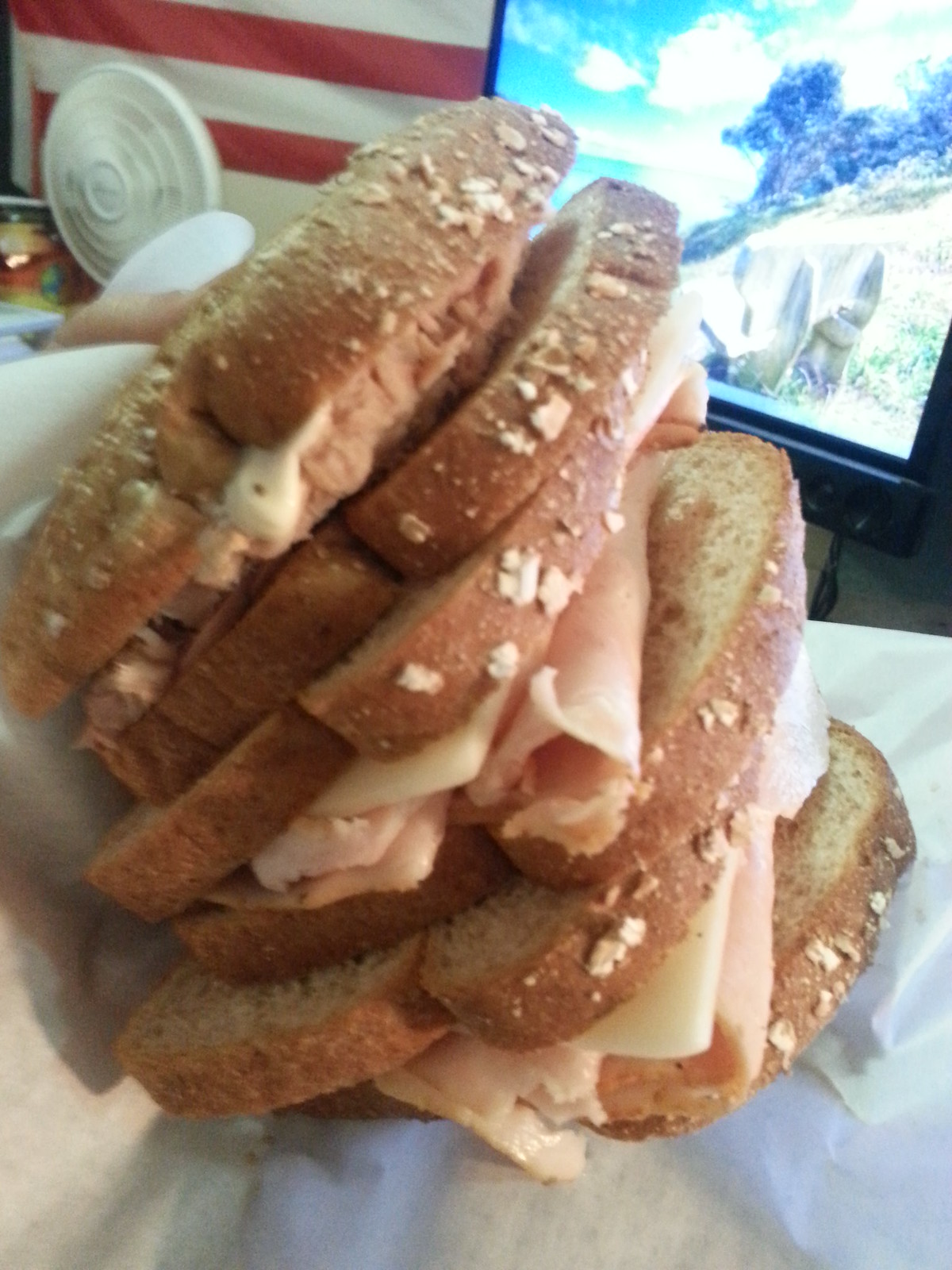In this photograph, three sandwiches are precariously piled atop each other on a white piece of paper. They are made from five slices of wheat bread with a golden brown crust, topped with oats or seeds, giving the bread a lightly crumbed and flaky appearance. Inside, the sandwiches contain processed lunch meat—like ham, turkey, or possibly shredded tuna—paired with a slice of white cheese, with the top sandwich showing a hint of mayonnaise. The sandwiches are leaning toward the left side, making the pile look haphazard. They rest on what seems to be a white countertop. The background features a black-framed TV or monitor in the top right, an American flag with red and white stripes to the left, a small white portable fan in the top left corner, and a silver tray or a cream-colored book in front of it.